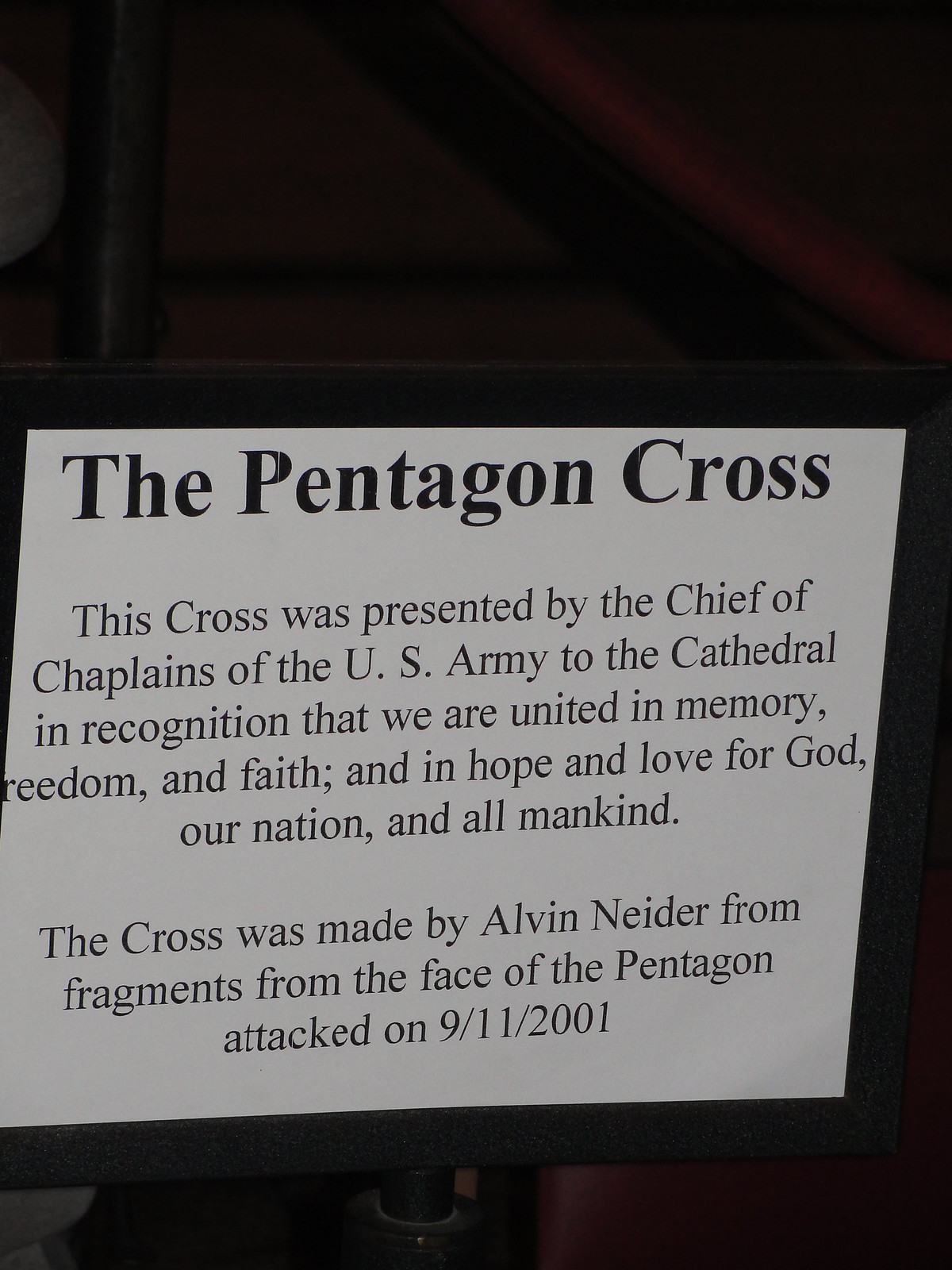This is a photograph of a white placard with black text, set against a black background. The placard is titled "The Pentagon Cross" in large, bold letters at the top. Below the title, the text reads: "This cross was presented by the Chief of Chaplains of the U.S. Army to the Cathedral in recognition that we are united in memory, freedom, and faith, and in hope and love for God, our nation, and all mankind." Additional spaced text at the bottom notes: "The cross was made by Alvin Nieder from fragments from the face of the Pentagon attacked on 9-11-2001." The placard appears to be attached to a hand railing.